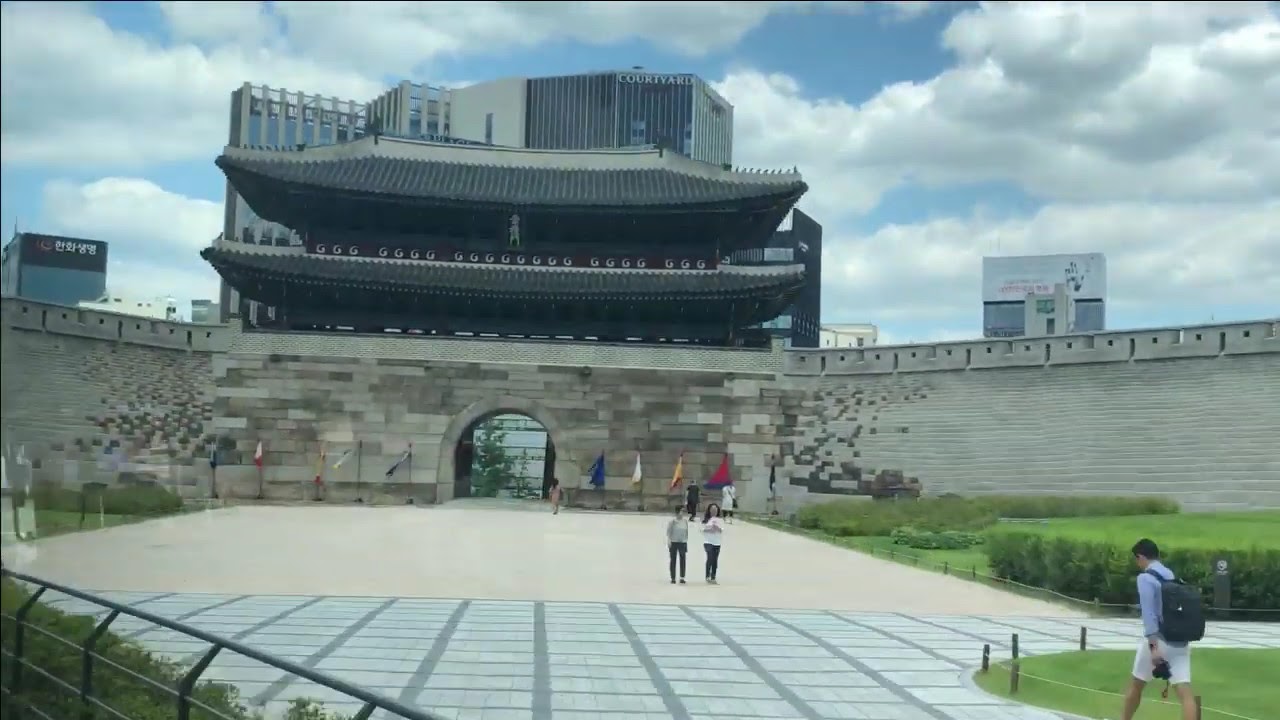The image depicts a vast, open courtyard leading to an impressive stone wall featuring a grand archway. The walkway in the forefront is composed of both stone tiles and smooth tan paving, transitioning to a wide expanse of white concrete. Carefully marked-off grassy areas line the walkway, bordered by low wooden stakes. The focal point is the monumental stone wall with an arched entrance, showing signs of wear and bearing five distinct flags—red, yellow, white, black, and blue. In the scene, a young man with white shorts, a blue shirt, and a dark backpack is seen walking away from the viewer, while two others approach on the broad walkway. Rising above the wall is a multi-storied, glass and steel building reminiscent of a pagoda style structure, flanked by two smaller edifices. In the background, towering commercial skyscrapers pierce the mostly cloudy daytime sky.